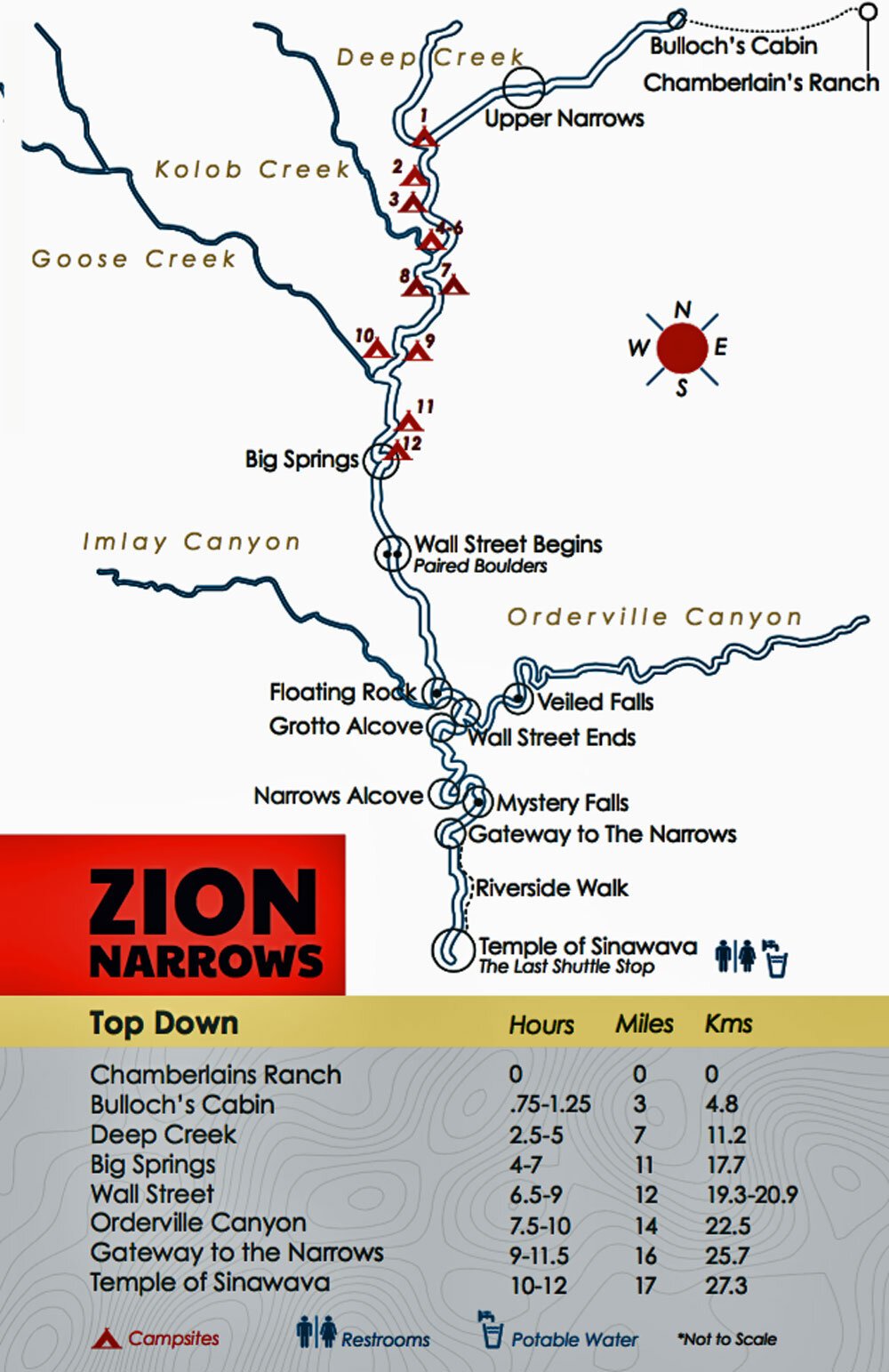This image depicts a detailed map of the Zion Narrows trail, characterized by various labeled locations and symbol indicators. The central map features multiple marked spots on the trail, with specific symbols indicating campsites (resembling tents), restrooms, and portable water sources. The map also includes a compass rose denoting northwest, east, and south directions.

Prominent texts and landmarks on the map include Deep Creek, Collab Creek, Goose Creek, Imlay Creek, Orderville Canyon, and a notable Zion Narrows logo in black text within a red box. Adjacent to the map, there is a gray section with a digital wood grain texture, labeled "Top Down," listing locations along the trail such as Chamberlain's Ranch, Bullock's Cabin, Deep Creek, Big Springs, Wall Street, Orderville Canyon, Gateway of the Narrows, and Temple of Shinawa. This list includes details with hours, miles, and kilometers to each point.

The bottom of the image distinctly categorizes the symbols for campsites, restrooms, and portable water, and explicitly notes that the map is not to scale.